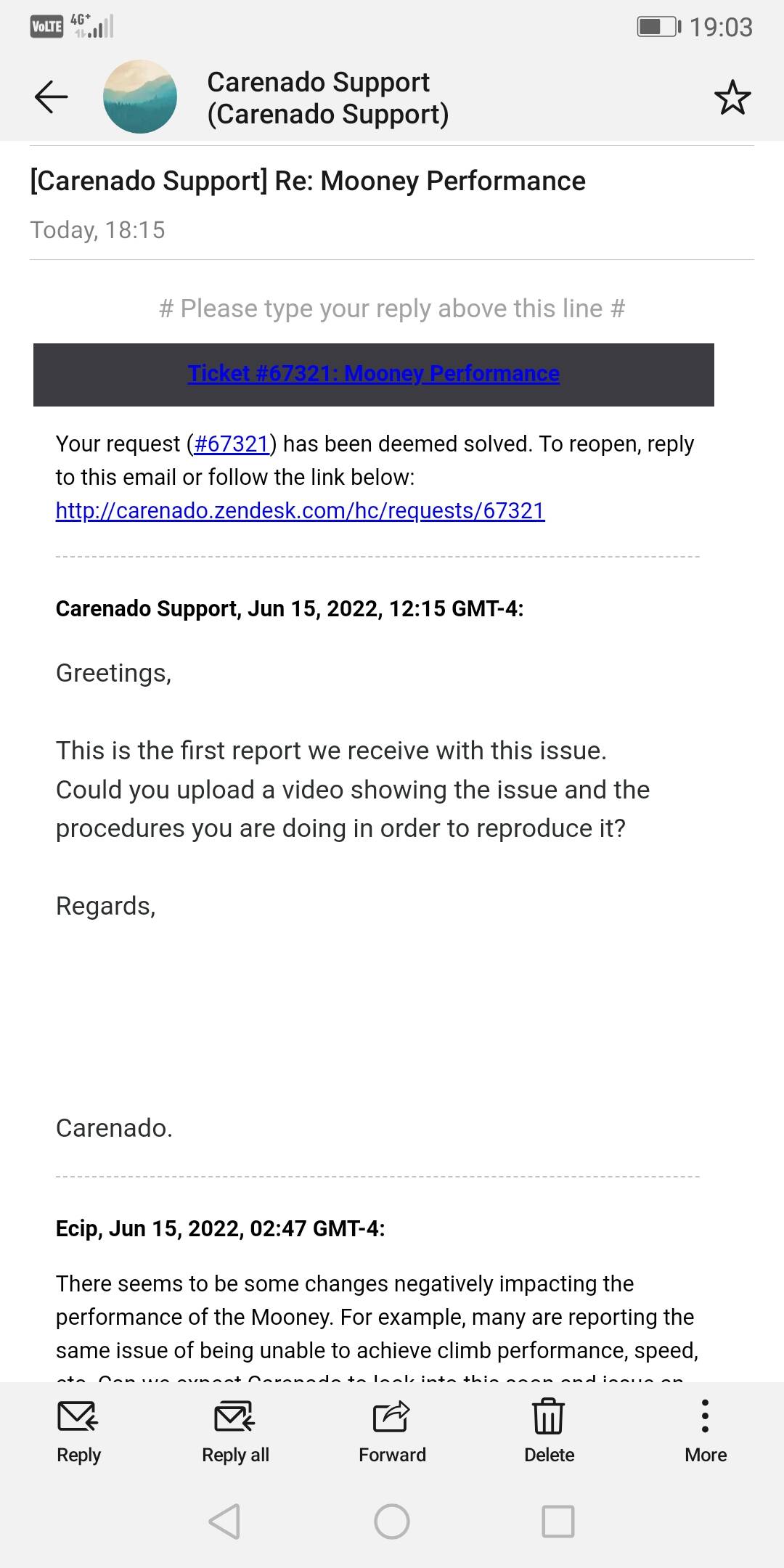The image depicts a screenshot from an email application, showing an email open on the screen. This email is from Carenado Support, which is part of the Carenado company, likely handling customer inquiries and technical support. 

The email displayed is a reply and is indicated in the subject line as "Carenado Support, reply, money performance." The timestamp below the subject line shows that this email was sent today at 8:15 PM. 

Central to the image, there is an instructional note in light grey text surrounded by two pound symbols (##) that reads, "please type your reply above this line." This suggests that the user can add their response directly above this line within the email. 

Just below the reply area, a segment of dark blue text is seen, though it is difficult to read clearly due to the dark grey background it blends into. The text appears to detail the ticket information related to this inquiry, stating, "ticket number 67321, money performance." 

The screenshot effectively captures the essential elements and structure of the ongoing communication between the user and Carenado Support regarding a previously raised issue.